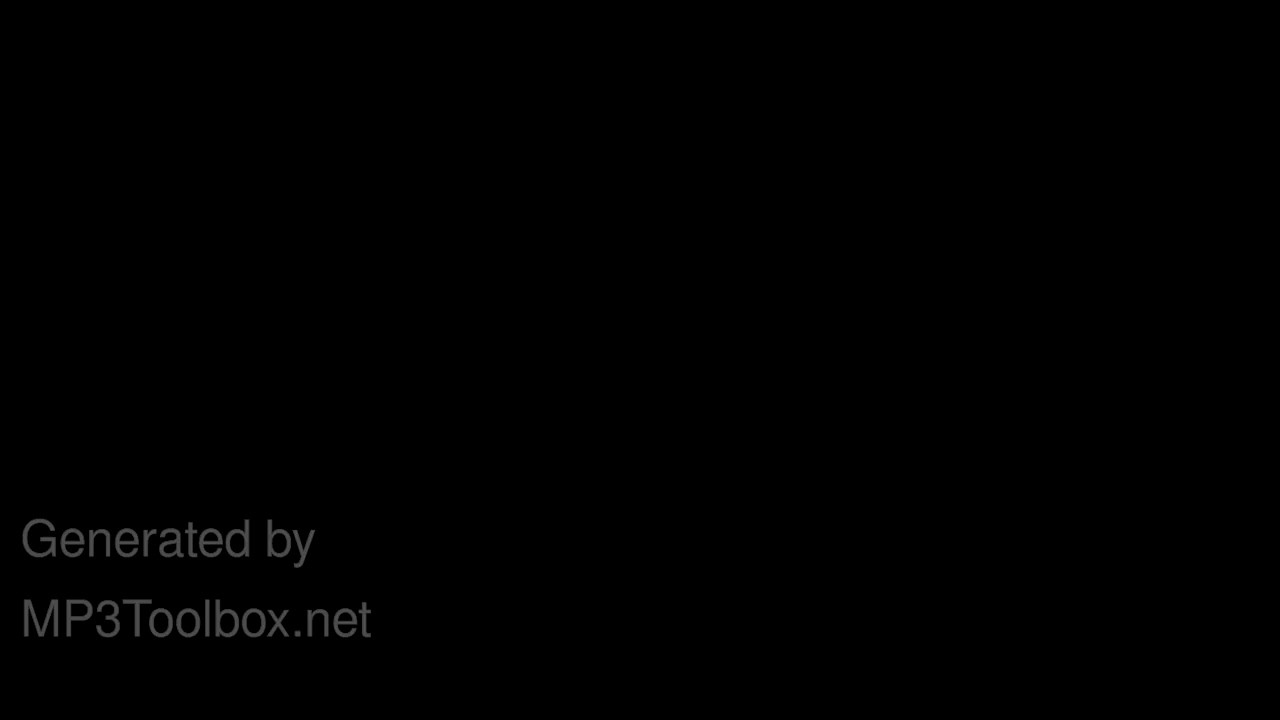This is a wide, rectangular image that is approximately twice as wide as it is tall. The background is a solid, pure black color with no objects or images present. The only content in the image is text located in the bottom left corner, written in a medium gray font. The text is relatively large but occupies a small portion of the image. It appears in two lines: the first line reads "GENERATED BY" with the 'G' capitalized, and the second line reads "mp3toolbox.net" with the 'M', 'P', and 'T' capitalized. The image seems very simple and minimalistic, potentially serving as a stock image.